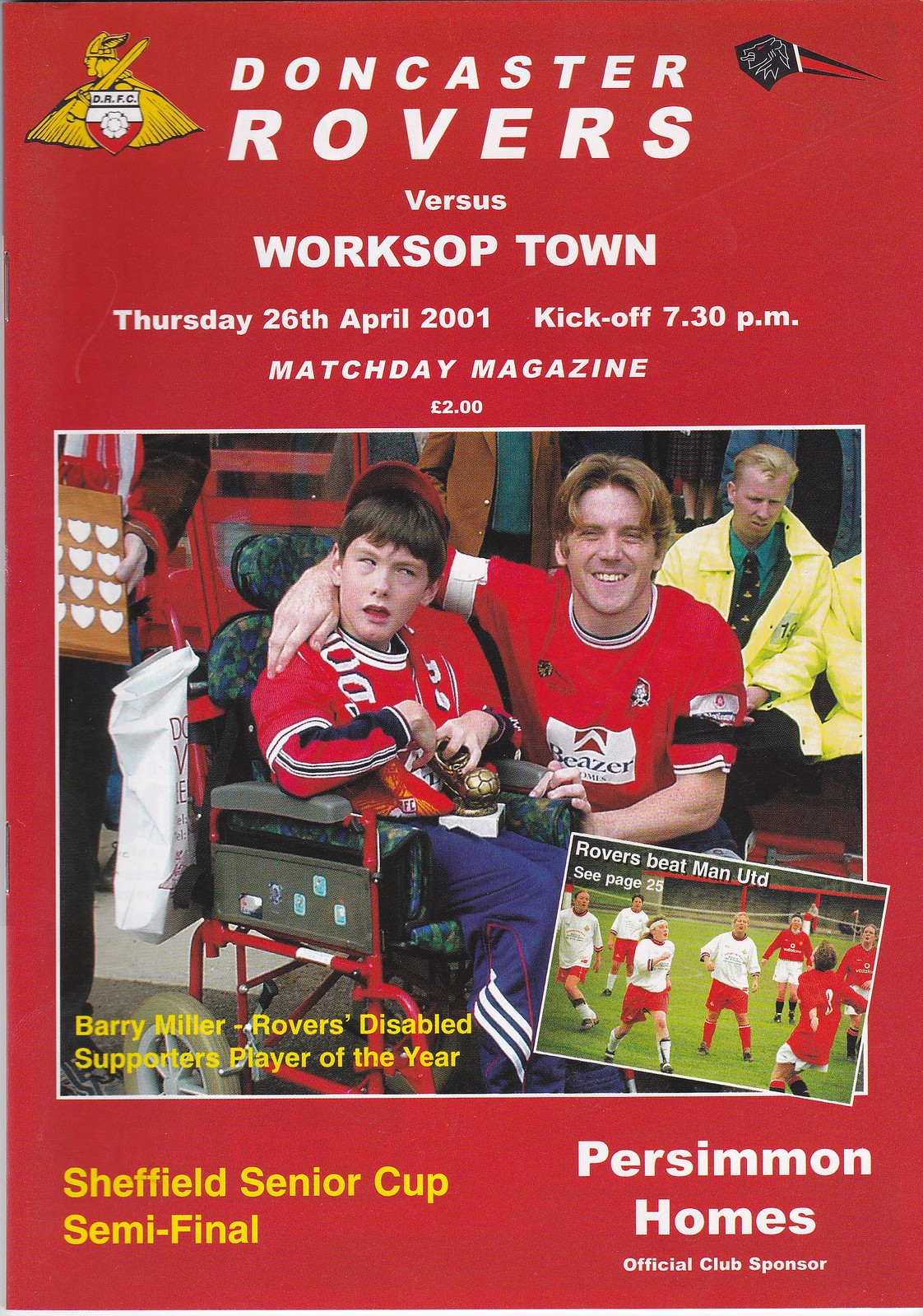The cover of the Doncaster Rovers match day magazine for the game against Workshop Town on Thursday, April 26, 2001, is striking with its bold red background. At the top left, the Doncaster Rovers Football Club (D-R-F-C) logo, featuring a yellow Viking in white text, catches the eye. The details of the event are prominently displayed: "Doncaster Rovers vs. Workshop Town, Thursday, 26th April 2001, kickoff 7.30 p.m.," followed by "Match Day Magazine, 2 lbs." 

Dominating the cover is a heartwarming image: a blonde soccer player in a red jersey kneels down, embracing a young boy in a wheelchair who also wears a red jersey and hat, along with blue pants. This touching scene is further accentuated by the text "Barry Miller, Rovers Disabled Supporters Player of the Year" in yellow at the bottom left of the image. In the background, spectators can be seen, some dressed in yellow slickers. Overlaying this main image is a smaller picture with the caption, "Rovers beat Man United, see page 25," depicting players in red and white uniforms on a green field.

Adding more context, in the bottom corners of the cover, additional text reads, "Sheffield Senior Cup Semi-Final" in yellow on the left, and "Persimmon Homes Official Club Sponsor" in white on the right. The layout and comprehensive detail make it clear that this is not just a magazine cover, but a commemorative piece capturing a significant event for the Doncaster Rovers and their community.